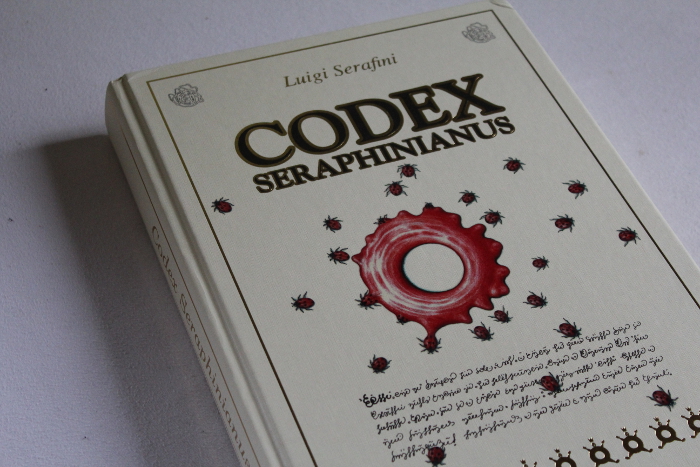The image features a white book laying diagonally at an angle from the upper left-hand corner to the lower right-hand corner of the frame against a clean, white background. The book itself, prominently centered in the image, bears the name "Luigi Serafini" at the top in golden lettering. Below that, in bold letters outlined in gold, it reads "Codex Seraphinianus." Central to the cover is an intricate artwork depicting a vortex of red liquid from which dozens of bugs appear to be crawling out. This vivid, detailed illustration is surrounded by additional small images, including what look like golden circular figures or turtles wearing crowns, potentially embroidered into the cover, and details such as flower petals in the upper corners. Below the artwork, the cover features handwriting resembling an ancient, unintelligible script. The book cover is framed by a thin black border. Colors in the scene include white, off-white, black, red, maroon, and gray. The setting seems to be indoors, possibly in a personal study or a library.